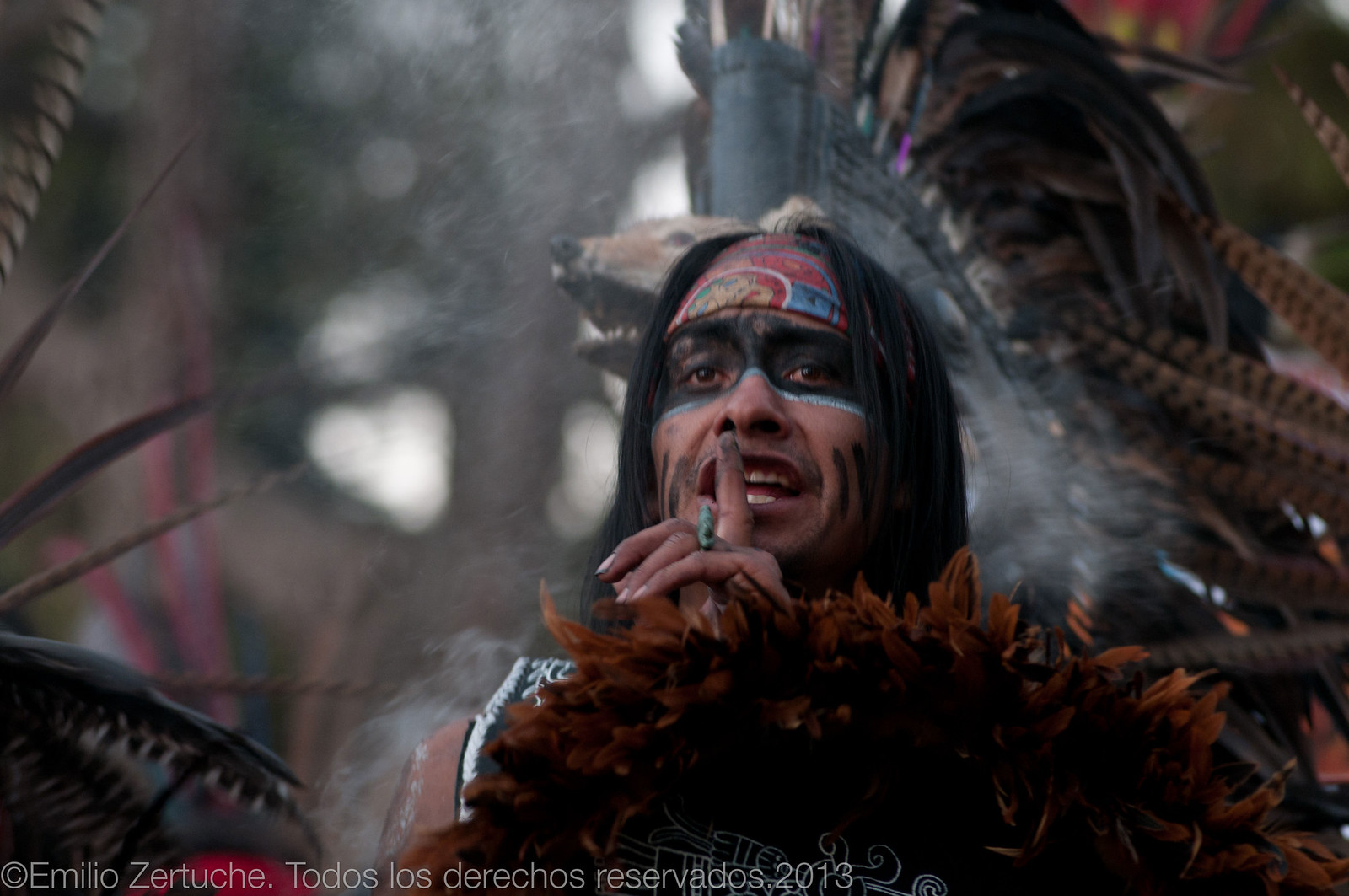This photograph captures an indigenous man, potentially from an Amazonian tribe, participating in a ritual. The man, with long black hair and black face paint prominently around his eyes, wears a headband and has a finger pressed to his lips, suggesting a gesture of silence. Feathers and what appears to be a stuffed fox head are visible behind him, adding to the ceremonial ambiance. Smoke swirls in the background, and the lighting suggests daylight, though it does not appear to be a particularly sunny day. The scene is set in a wooded area, with the man possibly crouching to blend into his surroundings. The colors in the image are predominantly earthy tones—browns, reds, and hints of white. In the bottom left corner, the text reads "Copyright Emilio Zertuche, Todos los Derechos Reservados 2013."